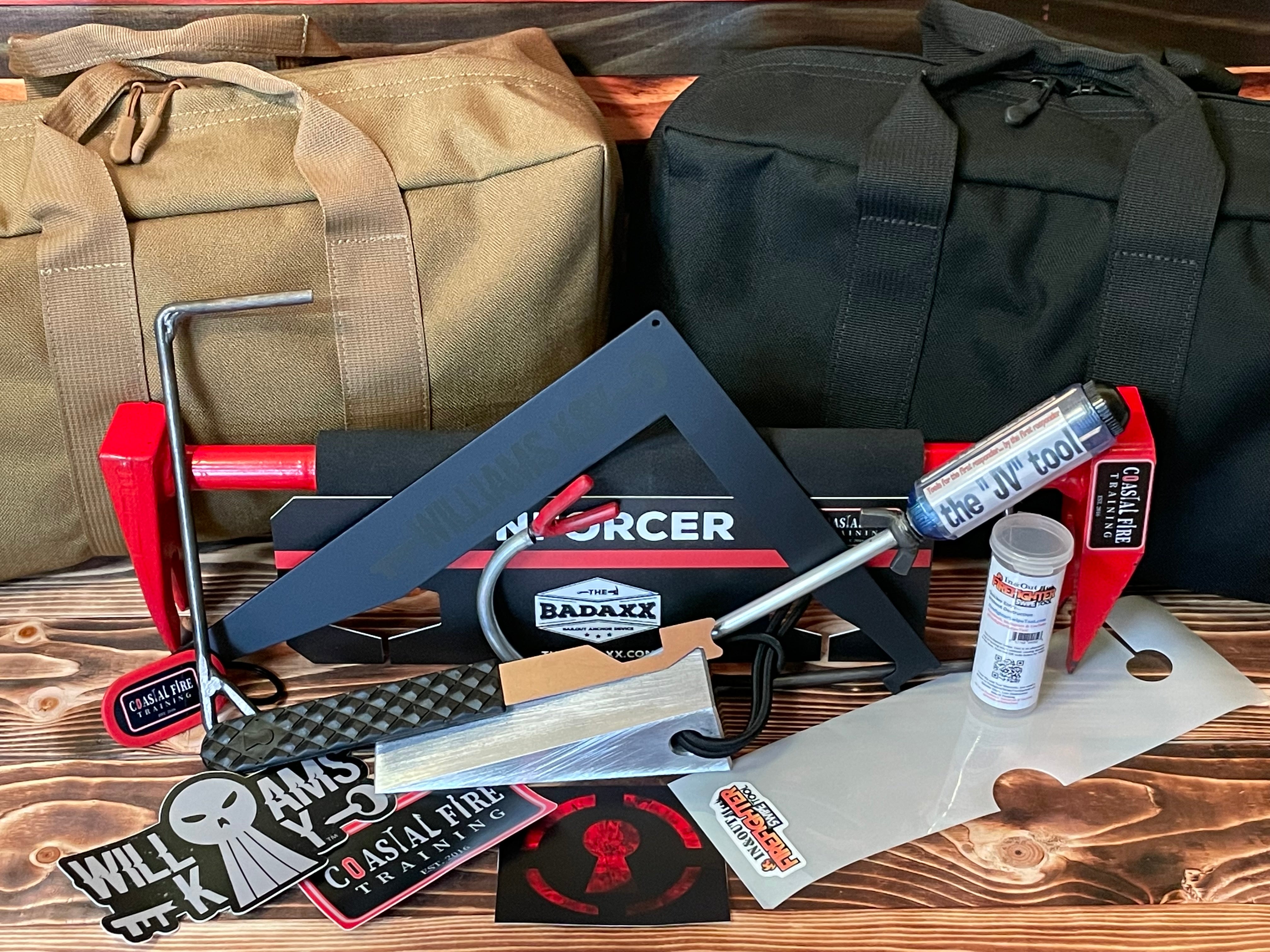The image showcases a detailed collection of tools and equipment meticulously arranged on a rich, wooden surface that features a prominent grain pattern, stained in contrasting hues of black and brown. Centered prominently are two distinct travel bags—a light beige duffel bag on the left and a black one on the right. Spread out in front of these bags is an array of predominantly firefighting tools, including a black L-shaped square bar, an angle bar, a chisel, a hammer, a saw, and a distinct red-colored axe likely used for breaking glass. Several tools are still encased in their original packaging, bearing labels and stickers from various manufacturers and vendors. The labels include "JV2," "Coastal Fire Training," "Williams Quay," and "Badax." Despite the diversity of items, the color palette remains cohesive with dominant shades of black, red, white, and brown. Overall, the image portrays a well-organized assembly of new, high-quality tools and equipment intended for professional use.